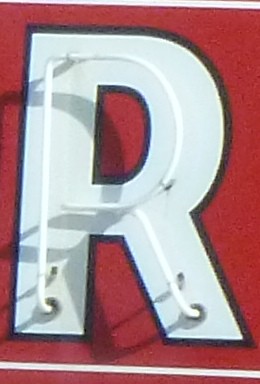The close-up image showcases a neon sign featuring a striking letter 'R.' The letter 'R,' prominently displayed in white with a black trim, is placed against a vivid red background. Inside the 'R,' neon lights form its shape, emitting a bright glow. The 'R' appears mounted with visible clamps where the neon tubing exits through various holes. Adding to the design, there's both a white stripe running across the top and another underneath, each bordered by additional red portions. This detailed and vibrant setup is typical of neon signs often found in windows, designed to attract attention with their illuminated features.